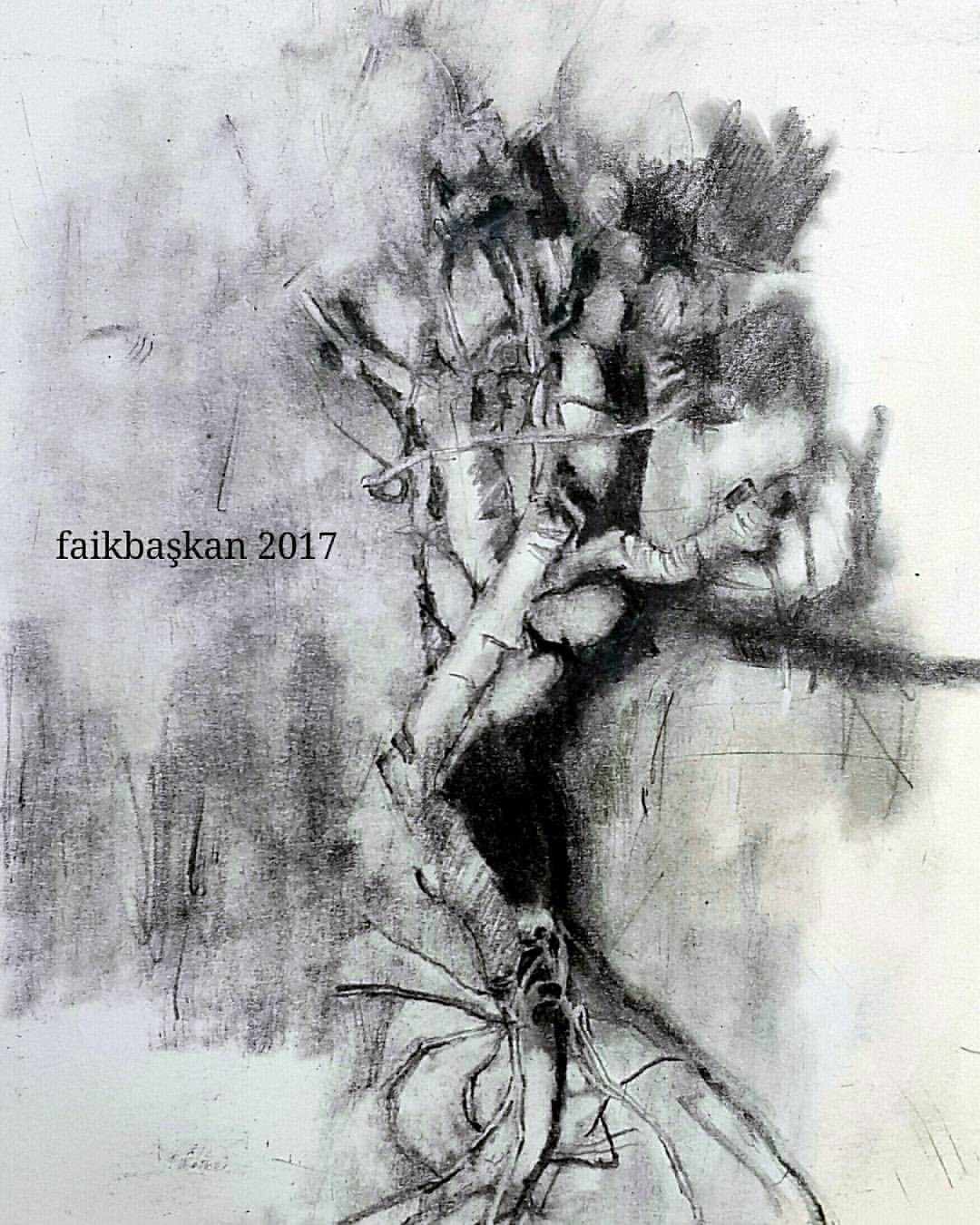This black and white charcoal drawing, titled "Thick Baskin 2017" as inscribed in the left middle of the artwork, presents an enigmatic and heavily shaded composition. Dominating the visual space, a twisted, tree-like figure rises from slender, root-like tendrils located at the bottom center of the image. The main structure, broad and white, ascends vertically before curving near the top. At this bend, it bifurcates into two additional thick, white branches, adding to the intricate and somewhat abstract nature of the piece. The overall aesthetic, marked by its heavy shading and complex forms, suggests a surreal and intriguing visual experience.